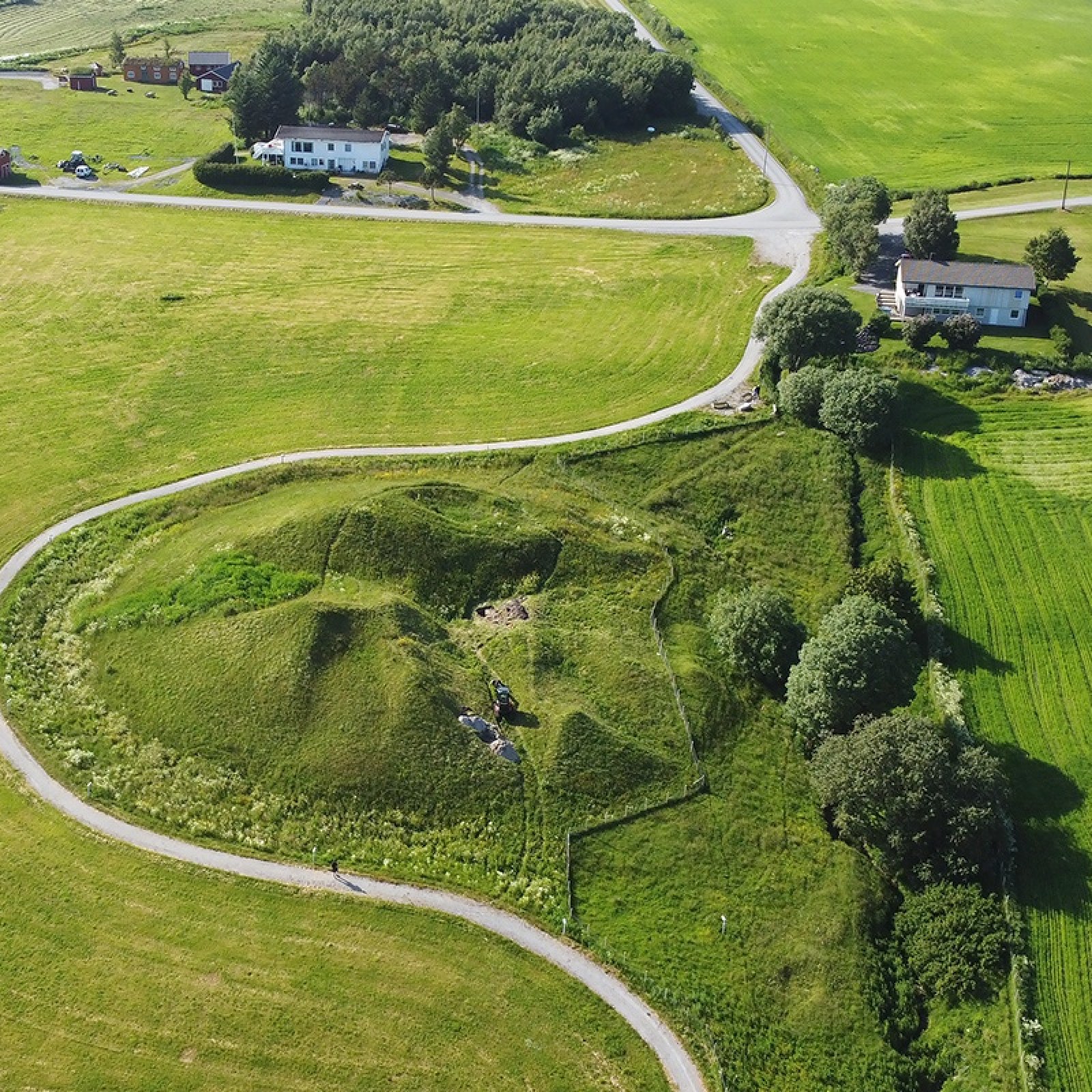The image is a professional overhead aerial shot, initially resembling farmland but more accurately depicting an extensive backyard area. Dominated by lush greens and patches of yellow hues, the scene highlights two distinct white houses with brown roofs, located towards the right side of the image. A sinuous walking trail, forming a U-shape, winds through the center of the picture, threading through a hilly area characterized by gentle rises and falls, covered in grass. The landscape is interspersed with various shades of green from the shrubbery and trees, complemented by scattered rocks. A vertical line of trees runs along the right side, and a horizontal road cuts across the picture near the houses. The lower left corner features an empty field of well-manicured grass, with no visible people, adding to the expansive and tranquil feel of the land. The daylight setting ensures a clear, detailed depiction of the vast area.